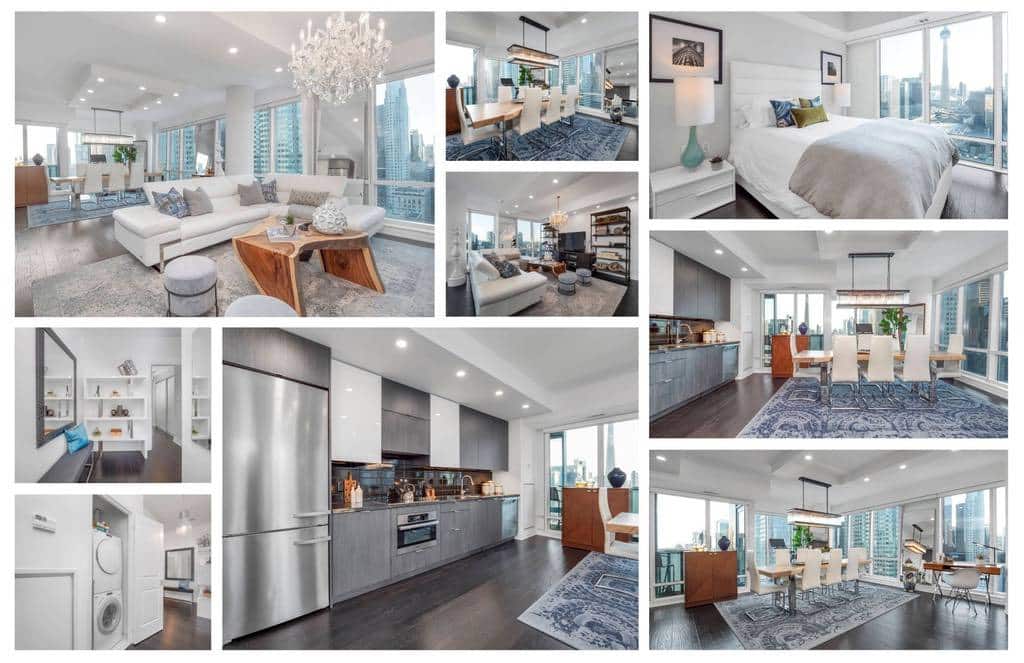The image is a horizontally rectangular collage showcasing various interior spaces of the same household. Each segment of the collage varies in size, from smaller square frames to larger horizontal rectangles, offering a comprehensive tour of the home. 

The kitchen is dominated by a modern aesthetic with stainless steel appliances and a color palette of gray and white, creating a sleek and contemporary feel. Adjacent to the kitchen, the expansive living room features a plush white couch and is illuminated by a sophisticated chandelier, casting a warm glow over the space.

The dining area is equally elegant, furnished with white high-backed chairs that surround a long dining table, perfect for hosting gatherings. In contrast, the bedroom exudes comfort and tranquility, highlighted by a large bed adorned with a white headboard, pristine white sheets, and a cozy gray comforter.

From one of the windows, there is a captivating view of a bustling cityscape filled with towering skyscrapers, suggesting that the household is situated in a highly populated urban area. This collage beautifully captures the modern and luxurious essence of the home, offering glimpses into each thoughtfully designed space.